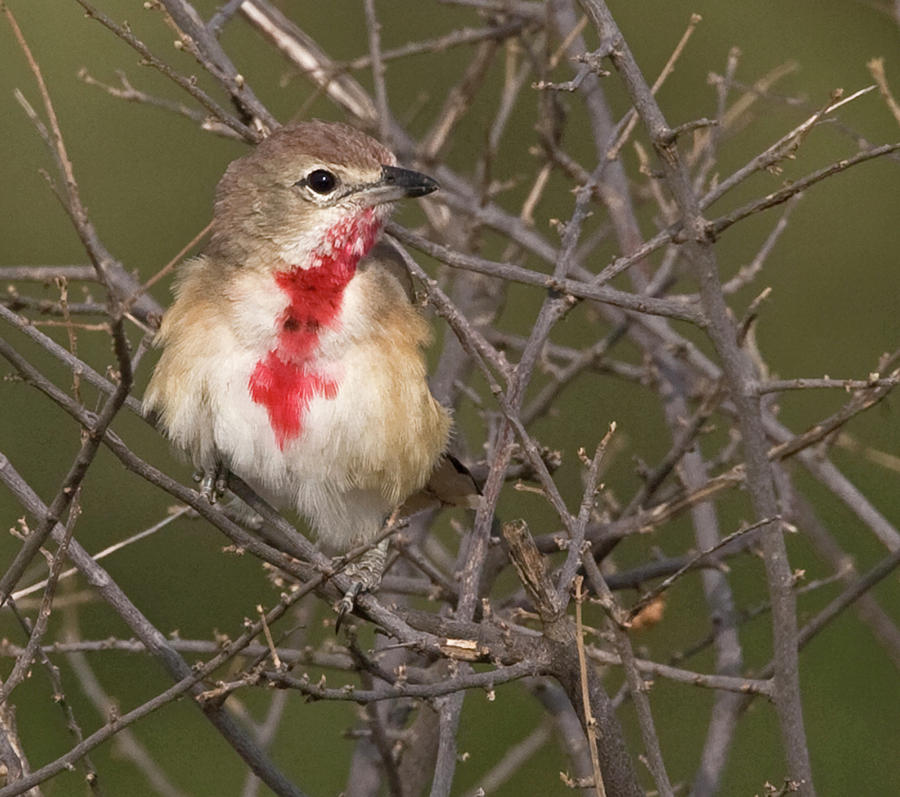The photograph captures a close-up scene of a small bird perched in a tree during the daytime. The bird, which resembles a miniature chicken in shape, features a white belly and a brownish head with a short black beak. Its crown and the back of its head also appear to be brown, transitioning to a lighter color at the front of its face. The bird's body is primarily white with hints of yellow. However, the most striking detail is a large, red stain that extends from below its beak to its chest, which appears to be either blood or remnants of something red it has encountered, possibly berries. Despite the unsettling presence of the stain, the bird looks calm and comfortable. The tree it is perched on consists of a chaotic tangle of thin, leafless branches, suggesting it might be winter. The background is a blurred expanse of green, keeping the focus on the bird and the intricate network of branches in the foreground.